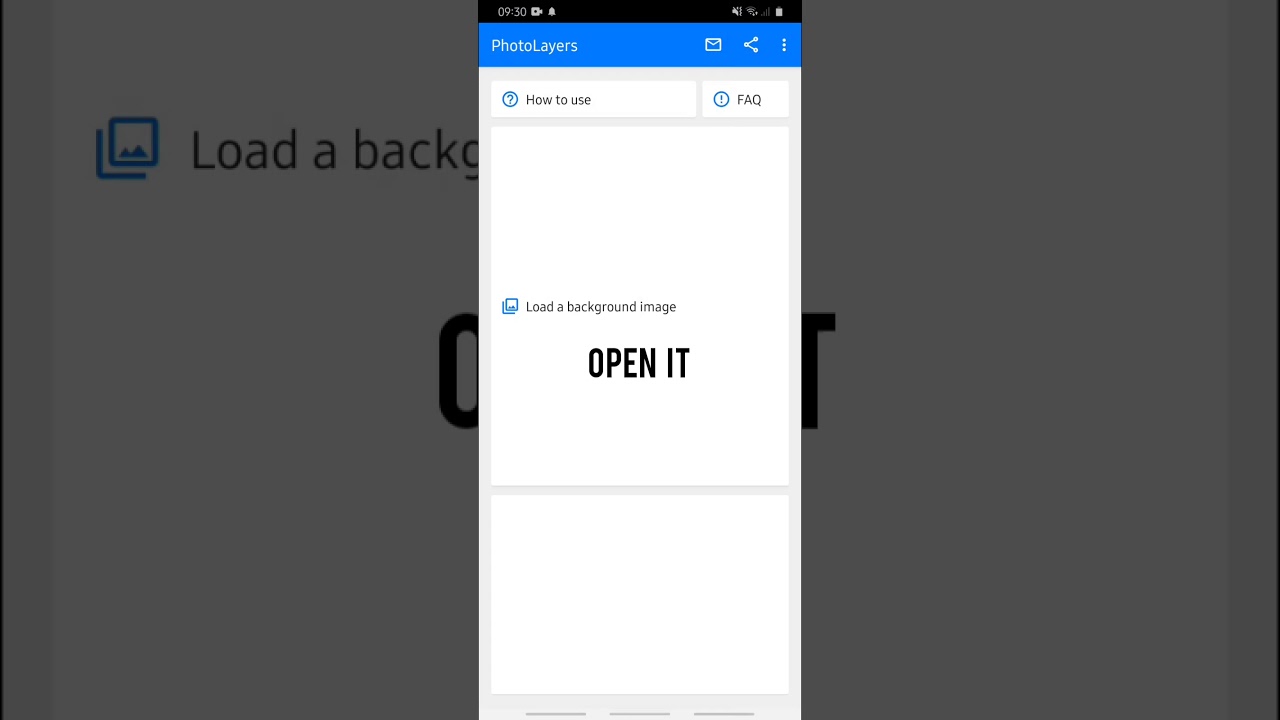This image displays a strikingly detailed user interface of a mobile application. Centered prominently on the screen, a large rectangular box with black text reads "Load a Background," though part of the word 'Background' is obscured under another element, leaving just "Load a Back" and a partial 'G' visible. This text is situated over a second rectangular box, which features the phrase "Open it" in all capital letters.

Superimposed on this main backdrop is a narrower, vertically oriented smartphone screen. This screen's header, set against a blue background, clearly reads "Photo Layers" in white text. To the right of this header, an icon resembling a share button (three linked dots forming an abstract 'V' shape) is shown, accompanied by a horizontal three-dot menu symbol.

Beneath the header, the vertical smartphone screen displays instructional and support options: "How to use?" marked with a question mark, "FAQ!" with an exclamation mark, and several other interface elements. Notably, under these options is a white box containing the phrase "Open it" in all capital letters.

The entire composition suggests a layered interaction, where actions taken in the vertical smartphone interface influence or modify the underlying larger background image. The preview seen in the image showcases how overlapping elements from the 'Photo Layers' screen align seamlessly with the visible portion of the 'Load a Background' prompt on the larger screen.